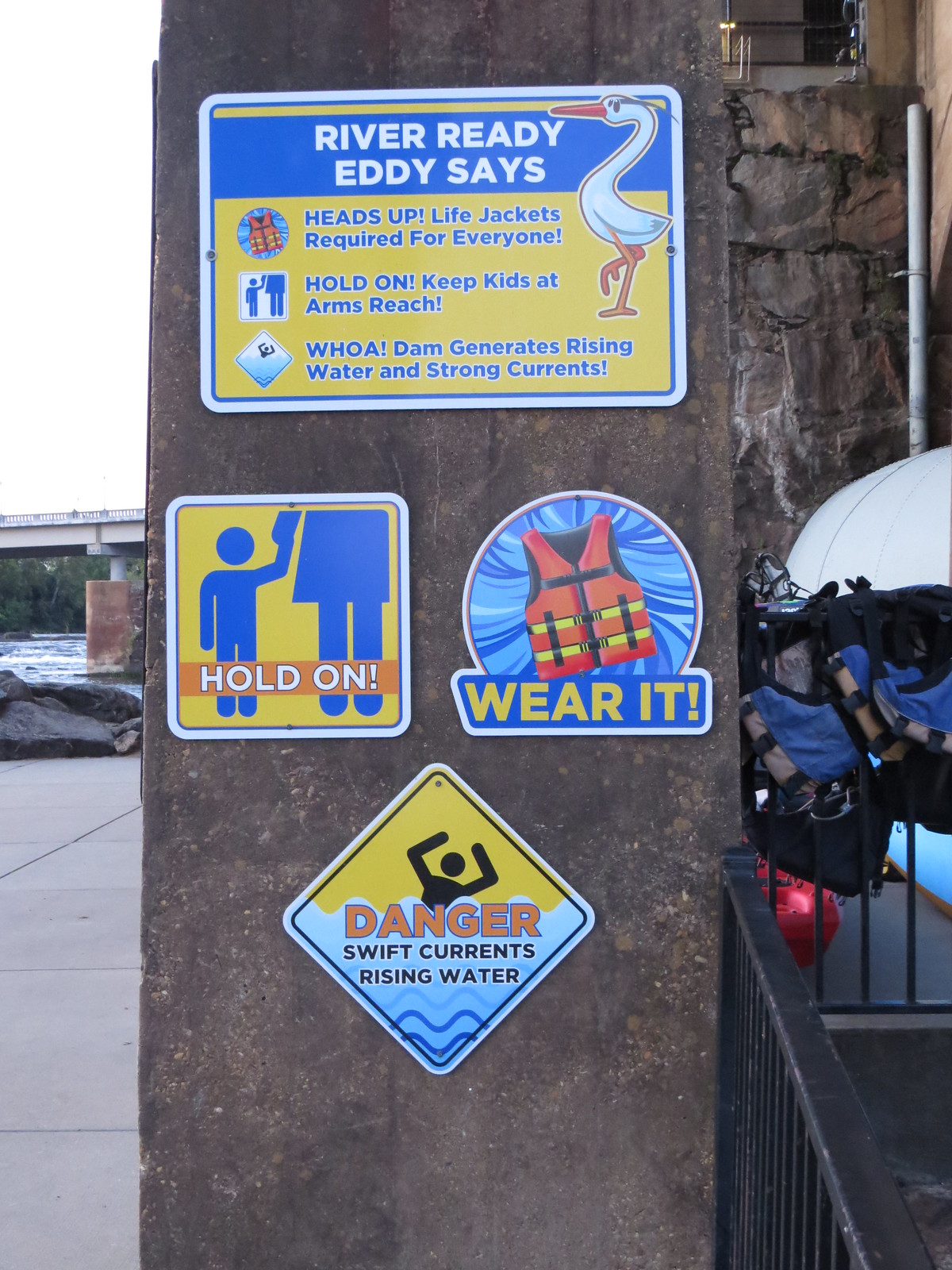In the image, we observe a dark brown pillar, possibly a rusted metal pole or stone column, positioned prominently in an outdoor setting beside a river. To the left of the pillar, several pieces of stacked stone are visible, with another dark brown pillar nearby, and a bridge crosses the river in the background. On the right side, a black metal fence stands with a lifejacket or some floating device resting atop it.

The pillar features four distinct signs. The top rectangular sign has a blue banner across its top and predominately yellow background detailing. It reads, "River Ready Eddie says," followed by "Heads up, lifejackets required for everyone. Hold on, keep kids at arm's reach. Whoa, dam generates rising water and strong currents," accompanied by an illustration of a stork or bird. Below this, two smaller signs convey safety messages: one square sign shows a child holding hands with a mother and states "Hold on," while a circular sign depicts a life vest with the words "Wear it" underneath. The bottom diamond-shaped sign depicts a figure in turbulent water with the message "Danger, swift currents, rising water." The signs are vivid with colors such as yellow, black, orange, and blue, emphasizing the important safety information for river visitors.